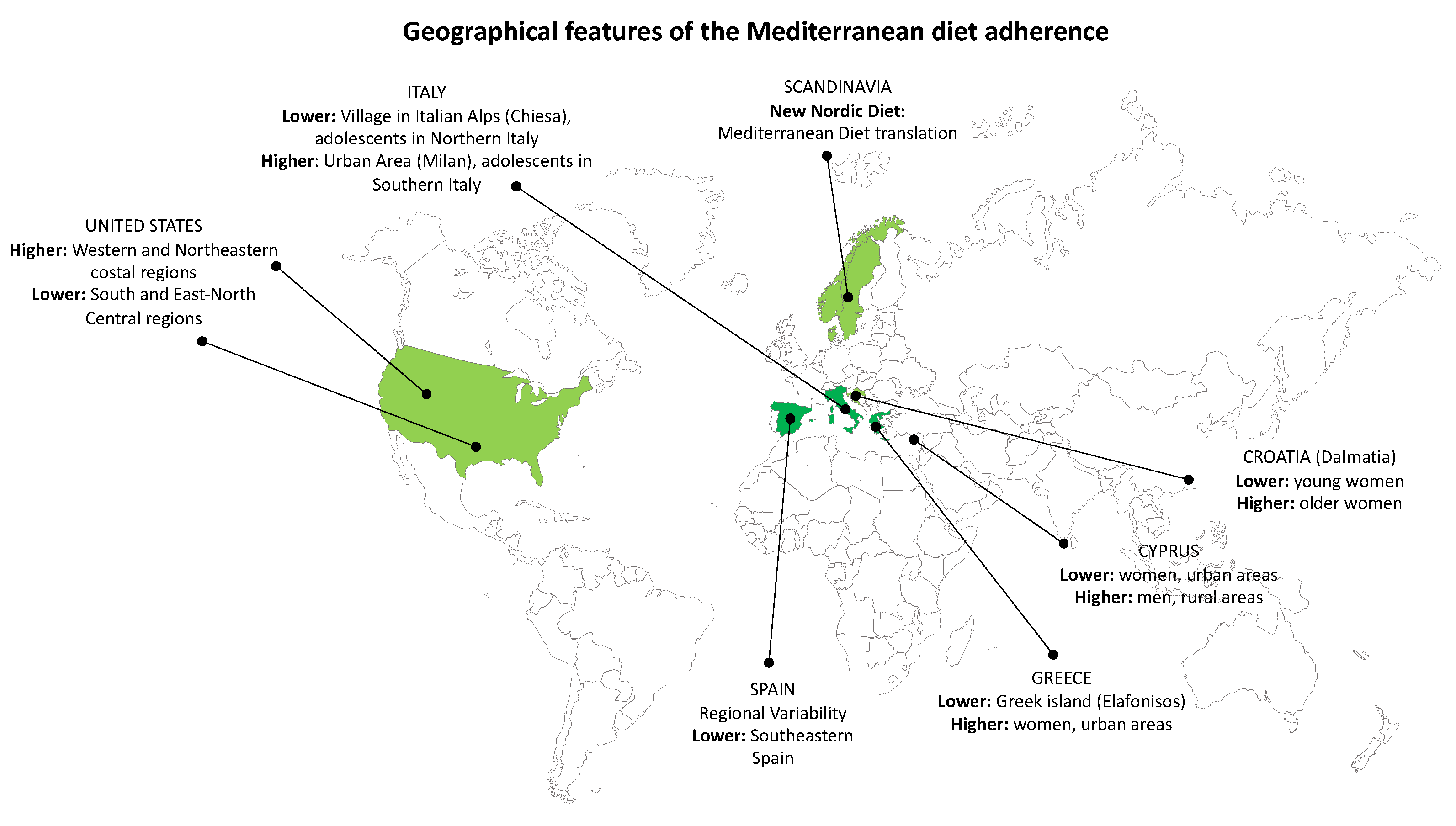The image, resembling a textbook illustration, displays a flat world map highlighting specific regions in various green tones to depict the "Geographical Features of the Mediterranean Diet Adherence” in black lettering at the top. Scandinavia and the United States are marked in lime green, noting dietary specifics: Scandinavia as the "New Nordic Diet Mediterranean Diet Translation," and the U.S. indicating "higher Western and Northeastern coastal regions, lower South and East North Central regions." In medium green, Southern European countries such as Italy, Spain, Greece, Cyprus, and Croatia are detailed with demographic dietary adherence: Italy highlights "lower village in Italian Alps, higher urban area Milan," Spain shows "regional variability, lower Southeastern Spain," Greece indicates "lower Greek island Elefthanesios, higher women urban area," Cyprus details "lower women urban areas, higher men rural areas," and Croatia marks "Dalmatia, lower young women, higher older women." Accompanying lines from each country provide concise demographic and geographical variances in diet adherence.